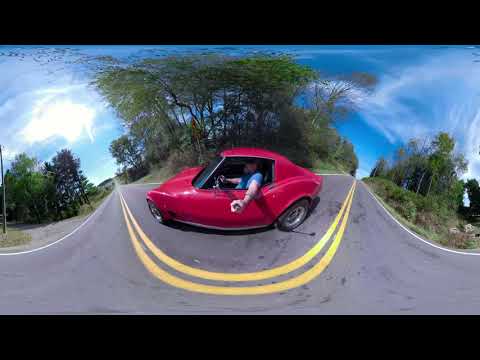The photograph captures a sunny day scene featuring a small, likely 1980s red car with no backseat, suggesting it is a two-seater or coupe model. The car, noticeably distorted due to the use of a panorama view or fisheye lens, is driving on the right side of a single-lane, two-way concrete road marked by a long, unbroken double yellow line creating a distorted U-shape in the image. Seated at the wheel is a white male driver, dressed in a blue t-shirt with his left arm casually hanging out of the window. The backdrop consists of an abundant green forest under a clear blue sky, indicating a summer afternoon. The setting has a European ambiance, inferred from the style of the car and the overall road construction.